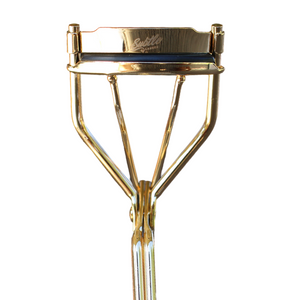This is a detailed close-up photograph of the top portion of a gold-colored eyelash curler against a plain white background. The image prominently features the upper section of the curler, with a particular focus on the crown-like design at the top. This design consists of two hands stretching outwards to connect the ends of the "crown," and two additional hands pushing up towards the middle. The top of the curler extends into a horizontally-oriented rectangular bar, which has a black, possibly rubber, strip for curling the eyelashes. The bar also features an etched logo or brand name in cursive lettering, though it is difficult to read. The shine of the gold metal is evident, with a reflective quality that shows some silver undertones where the gold appears to have scratched off. The lighting in the photo appears to come from the left, enhancing the visibility of these details. The handle of the curler is only partially visible, emphasizing the top portion of the tool in what looks like a professionally taken product photo intended for retail display.